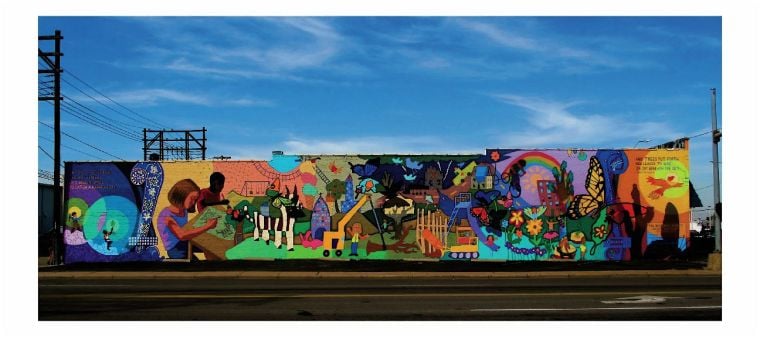This image captures a vibrant and intricate outdoor mural painted on the side of a building under a clear blue sky with a few light clouds that appear almost smoke-like. Power lines strung between wooden poles stretch across the scene, both on the left and right sides, leading to a large brown base in the background. Below the sky and wires, an empty road runs in front of the mural.

The mural itself is an explosion of bright colors and detailed imagery. On the left side, set against a purple background, is a blue circle featuring a person holding a torch. Next to this, there is a scene where two children or perhaps a man and a woman are sitting at a table drawing. This transitions into a scene where a construction vehicle is lifting a fallen tree. Further along, the mural depicts several flowers blossoming next to a fence, and a large monarch butterfly can be seen fluttering nearby. Additionally, there is a desert scene with a cactus silhouetted against what looks like a sunset. Adding to the richness of the mural, midway through is a depiction of a sugar cone with three scoops of ice cream.

This mural is surrounded by an environment that includes scattered, detailed elements such as monarch butterflies, a road sign with an arrow pointing to the right for upcoming turns, and some undetermined graffiti which is artistically expressive. Together, these elements create a lively and multifaceted scene, full of life and artistic celebration.